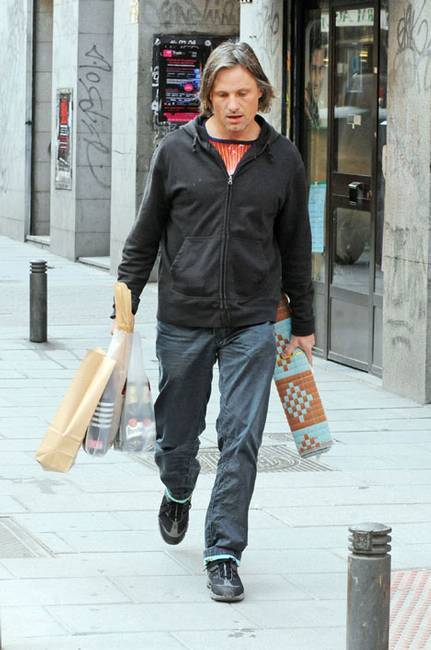A man is walking down a sidewalk in an urban area, caught in what appears to be a candid or paparazzi-style photo. He is wearing black shoes, gray pants or jeans, a zipped-up black hoodie with the hood down, and a vibrant orange-red shirt beneath. He has chin-length, unkempt hair and is clean-shaven. In his left hand, he is carrying a rolled-up item that resembles a throw rug or mat with a patterned design in white, tan, and possibly orange. His right hand is holding three bags—a paper bag and two plastic bags. One of the plastic bags clearly contains a six-pack of bottled beverages, and the other appears to hold some cups. The background features a mix of urban elements: brick buildings with graffiti, a storefront with a door he may have just exited, and cement columns also adorned with graffiti. There are various urban fixtures, including traffic-limiting posts on the sidewalk. The man is looking down at the ground as he walks, adding a sense of introspection or distraction to the scene.